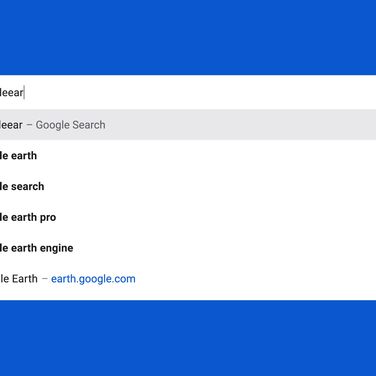The image is visually divided into sections with distinct elements:

1. At the top, there is a dark blue border running horizontally across the width.
2. Beneath this border, the central portion of the image features a white background.
3. In the upper part of this white area, there lies a text box that is partially obscured, making it difficult to fully discern its contents.
4. Prominently displayed within the white background is a Google search bar, which contains the partially typed letters "L-E-E-A-R".
5. Below the search bar, there is a highlighted area, broad in width but short in height.
6. This highlighted section features the text "L-E-E-A-R" followed by "Google search”.
7. Further down, a list of auto-suggestions on the white background includes:
   - L-E-Earth
   - L-E-Search
   - L-E-Earth Pro
   - L-E-Earth Engine
   - L-E-Earth Dash
8. Each suggestion is separated by a blank line.
9. Additionally, the text "earth.google.com" appears as a blue hyperlink among the suggestions.
10. At the very bottom, matching the top of the image, is another dark blue horizontal border.

This descriptive caption encapsulates all visual elements and the layout presented in the image.